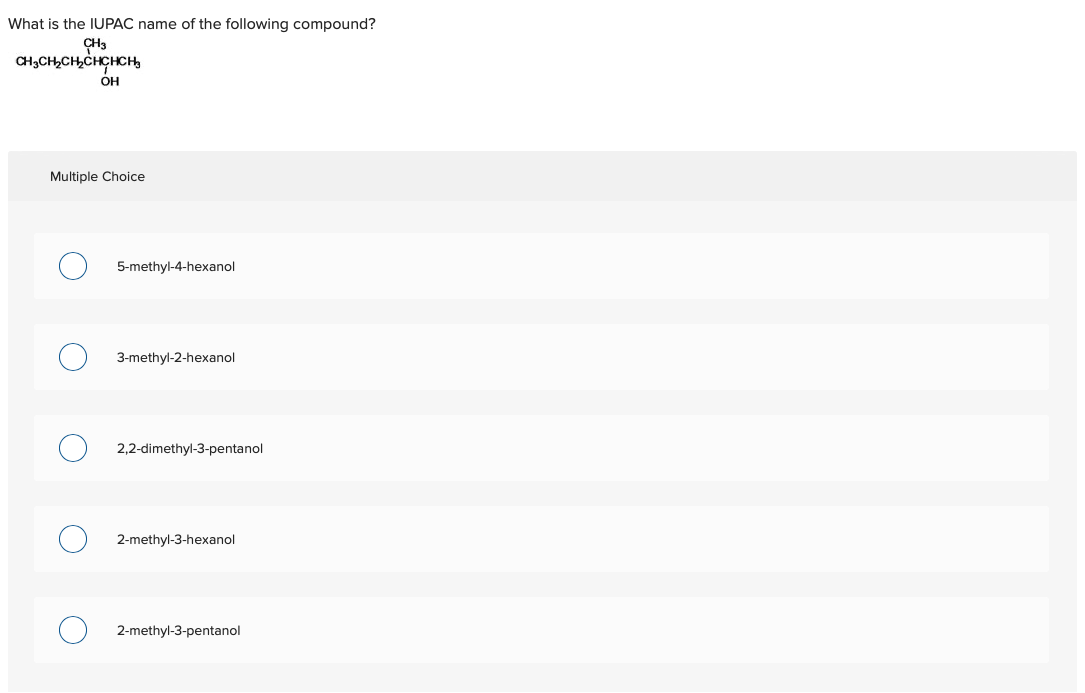The screenshot captures a partial view of a website featuring a chemistry question. At the top-left corner, there is a small black text reading, "What is the IUPAC name of the following compound?" The text "IUPAC" is notably in all caps. Below this question, a skeletal chemical structure of a compound is displayed. The main carbon backbone of the compound is depicted as a horizontal line, with two branches. One branch extends upward, labeled "CH3," indicating a methyl group. The other branch points downward and is labeled "OH," indicating a hydroxyl group.

At the bottom of the screenshot, a gray box titled "Multiple Choice" presents six possible answers for the IUPAC name of the compound:
1. 5-methyl-4-hexanol
2. 3-methyl-2-hexanol
3. 2,2-dimethyl-3-pentanol
4. 2-methyl-3-hexanol
5. 2-methyl-3-pentanol

None of the multiple-choice options have been selected, as indicated by the blank state of the corresponding bubbles. The surrounding background of the website is white.